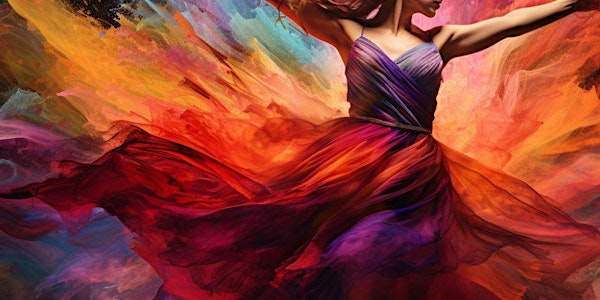In this captivating and colorful portrait, a woman is captured from her chin down to her mid-calves, set against an abstract, multicolored background bursting with shades of purple, aqua, dark reds, oranges, yellows, and blues. The woman, a brunette with only her lower face visible, is wearing a sleeveless dress with spaghetti straps. The main body of her dress is a blend of purple shades, transitioning into a flowing, gauzy skirt adorned in reds and oranges that create an illusion of flames or a fire dancer's attire. She has an orange, gauze-like fabric tied around her waist that undulates with her movement, adding to the dynamic, swirling effect of the image. Her arms are extended upwards, making her appear as if she's twirling gracefully amidst the vivid, painterly strokes of the rainbow-esque background. The overall effect is reminiscent of a sky painted in myriad colors, capturing the viewer's imagination with its ethereal beauty.